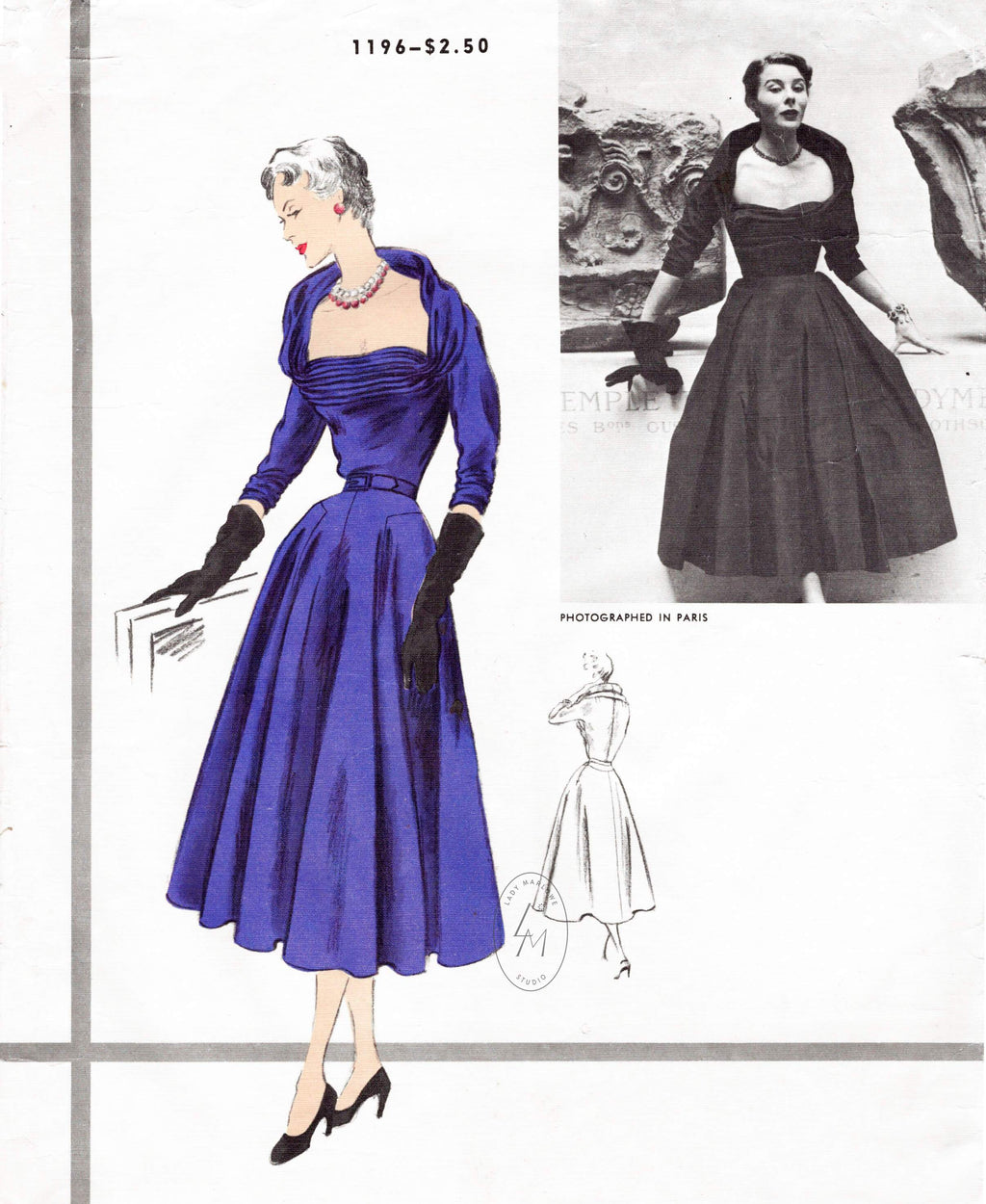This is a detailed Vogue advertisement from the 1950s showcasing a couture evening dress pattern priced at $2.50, designated as number 1196. The advertisement features both an illustration and a photograph. The main illustration depicts a woman in a royal blue ball gown with a cinched waist and a full skirt, paired with black elbow-length gloves, black high-heeled shoes, red lipstick, and red earrings. She accessorizes with a string of pearls and a necklace of red beads, and sports a short hairdo. 

Next to this illustration, there is a black and white pencil sketch showing the back view of the dress, highlighting its elegant design from all angles. Additionally, an inset black and white photograph of an actual model wearing the same dress is included. The model is depicted with one glove removed, leaning against a wall adorned with antique stone pieces, suggesting a museum-like setting. Her attire is complemented by black pumps and a clutch purse. This advertisement beautifully captures the fashion aesthetics of the 1950s, blending detailed illustration with real-life photography to entice potential buyers.